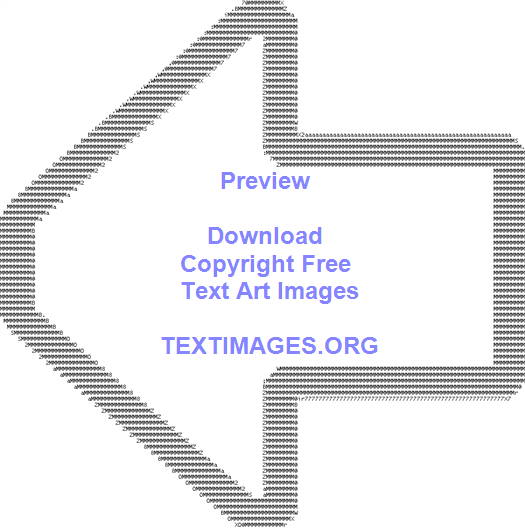The image features a large, bold arrow pointing to the left. The outline of the arrow is meticulously crafted from an assortment of letters, and possibly numbers or punctuation marks, creating a textured effect that requires close inspection to discern individual elements like O’s, X’s, and question marks. The arrow is primarily black, with a white interior. Centrally positioned within the arrow is a series of bold, light blue and purple text, which reads: "Preview." Beneath the word "Preview," the text continues with: "Download, Copyright-Free, Text Art Images," followed by "textartimages.org." The background of the image is completely white, accentuating the detailed design and boldness of the arrow. There are no people featured in this image, just the intricately outlined arrow with its informative text.